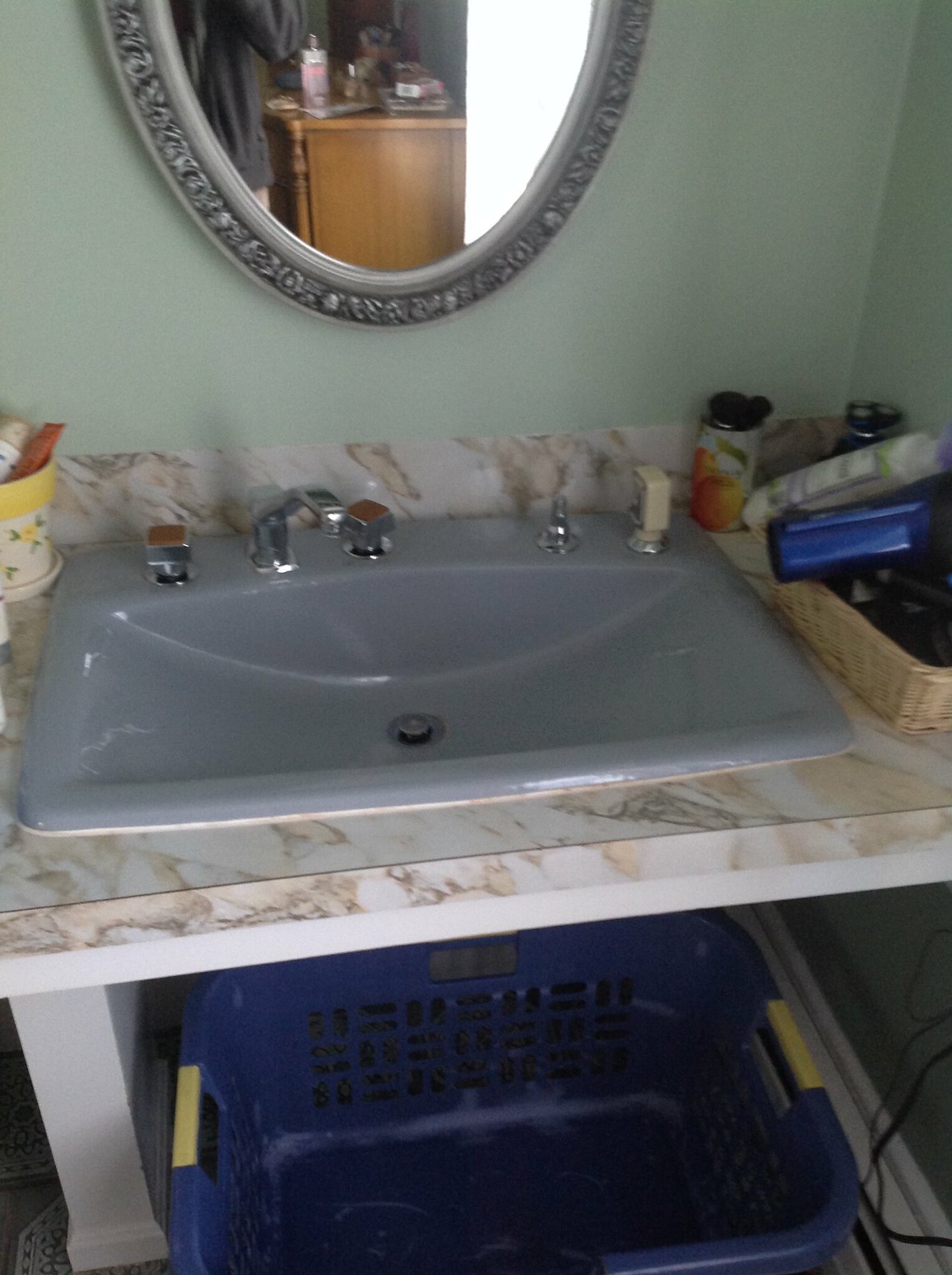This photograph showcases a meticulously organized bathroom vanity. Central to the image is a ceramic basin in a light grayish-purple hue, accompanied by chrome tap fixtures positioned to one side. The basin is set within a laminate benchtop, styled to mimic the appearance of marble. To the right of the basin, there is a straw basket filled with personal care items, with additional dispensing pumps visible behind the basket.

The wall in front of the vanity is painted a pale blue, complementing the overall aesthetic. An oval-shaped bathroom mirror with an engraved pewter-colored frame adorns the wall, adding a touch of elegance. The mirror's reflection reveals a brown cabinet, likely a chest of drawers, topped with a bottle of shampoo and partially obscured by the person taking the photo, who is wearing a black long-sleeve top with their face out of view.

Below the vanity, a hollow space houses a practical blue plastic basket featuring a vibrant yellow handle, highlighting the blend of functionality and style within this bathroom setting.